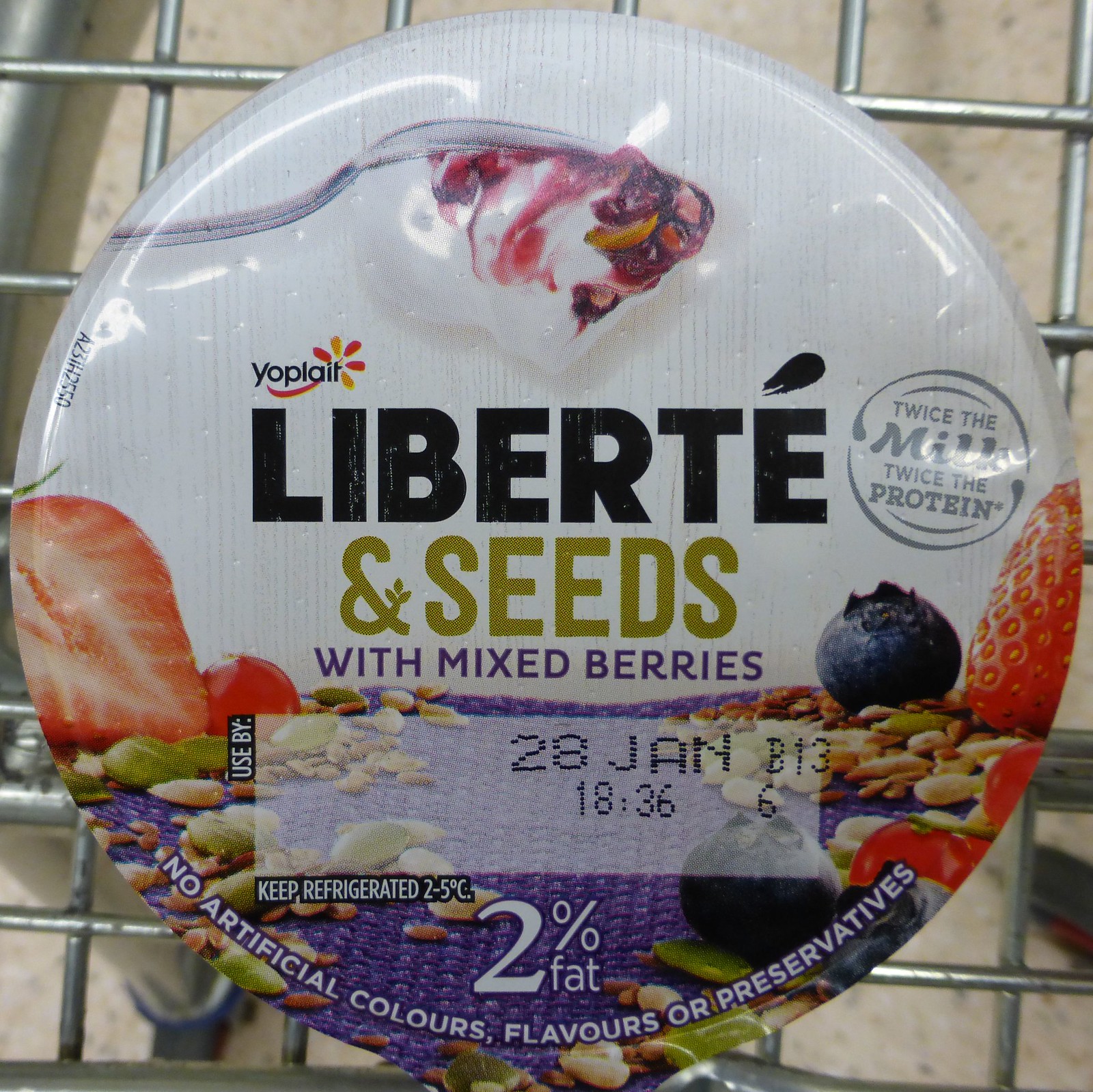This image showcases a close-up of the circular lid of a Yoplait Liberté yogurt container, resting at the top of a shopping cart. The lid predominantly features a white background with an upside-down spoon dipped in thick yogurt mixed with a red, fruity flavor, likely mixed berries. The Yoplait logo is prominent, adorned with red and orange flower motifs. The word "Liberté" is spelled with an apostrophe, in black font, while "Seeds" appears in a tan-brown hue. The lid also states "2% fat," "twice the milk, twice the protein," and assures "no artificial colors, flavors, or preservatives." Surrounding the spoon are vibrant images of strawberries, nuts, and blueberries, accentuating the mixed berries label. At the bottom of the lid, the expiration date "28 Jan" and the time "18:36" are stamped alongside the reminder to keep the product refrigerated. The image is set against the silvery metal bars of the shopping cart, with the grid-style pattern visible beneath the yogurt container.